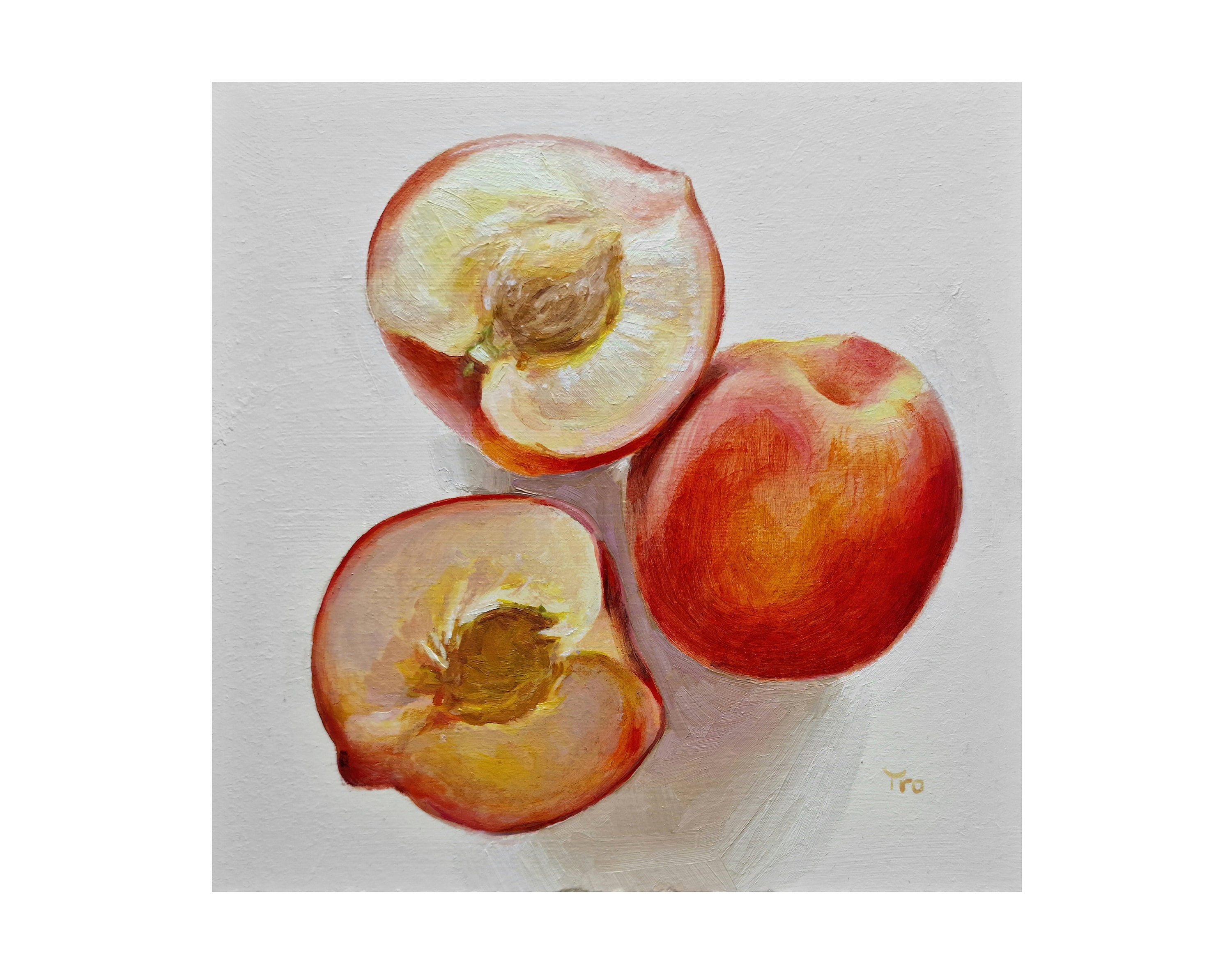The image is a detailed and vibrant oil painting of peaches. It features one whole peach with a red, orange, and yellow exterior, indicating its ripeness, alongside two peach halves. The insides of the halves display a fleshy, off-white to yellowish hue. One of the peach halves reveals a large, beige pit that is notably bumpy and intricate. The peaches in the painting look perfectly ripe and delicious. The artist has signed the artwork at the bottom right-hand side with the initials "T-R-O."